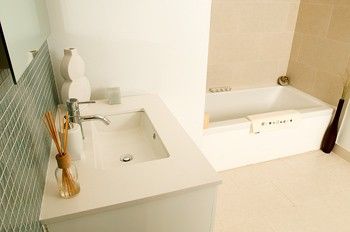The photograph captures a bathroom scene with distinct elements on either side. On the right side of the image, the bottom section features a tan-colored tiled floor. Above the floor, occupying the right side, is a rectangular white ceramic bathtub. Draped over the edge of the tub is a bath mat, and perched on the edges are some items, possibly a candle or soap container. The bathtub is set against a wall adorned with matching tan tiles.

On the left side of the image, we have a standard white rectangular sink with a marble-like finish, complemented by a metal faucet. On the top left corner of the sink rests a reed diffuser, commonly used for essential oils. Next to the diffuser is a soap dispenser. In the top right corner of the sink lies a tall, unidentified white object that reaches higher than the faucet. The upper left part of the image reveals the bottom portion of a mirror, completing the overall layout of this bathroom scene.